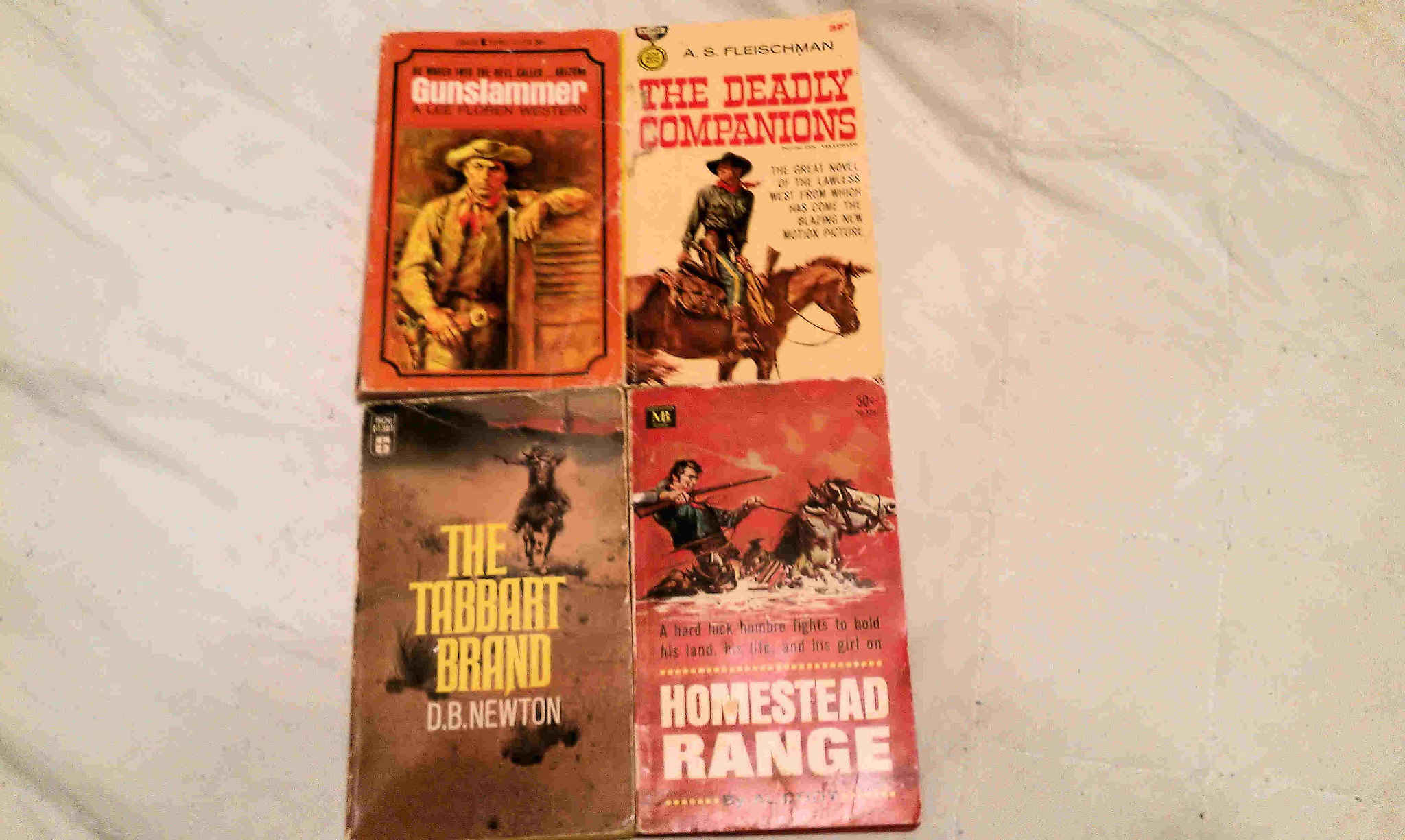The photograph showcases a collection of four vintage paperback Western novels arranged in a neat square on a wrinkled, white sheet background, likely taken on a bed. Each cover features illustrated depictions of iconic cowboy scenes. The top-left book, titled "Gun Slammer," has a red background with a cowboy clad in tan bursting through saloon doors, titled in white lettering. Adjacent to it on the top-right, "The Deadly Companions" by A.S. Fleischman features a tan background with a cavalry man on horseback, dressed in a green uniform, complete with a matching hat and side arms, with the price visibly stamped in cents, indicative of its age. The bottom-left book, "The Trabert Brand" by D.B. Newton, is set against a brown cover, showing a black horse charging forward with a rider in mountainous terrain, emphasized with a yellow title font. Finally, the bottom-right book, "Homestead Range," also with a red background, depicts a cowboy on a horse wading through deep water, holding a long rifle pointed to the right. Despite some blurriness and glare, the intricate details and themes of these old Western paperbacks are vividly brought to life.